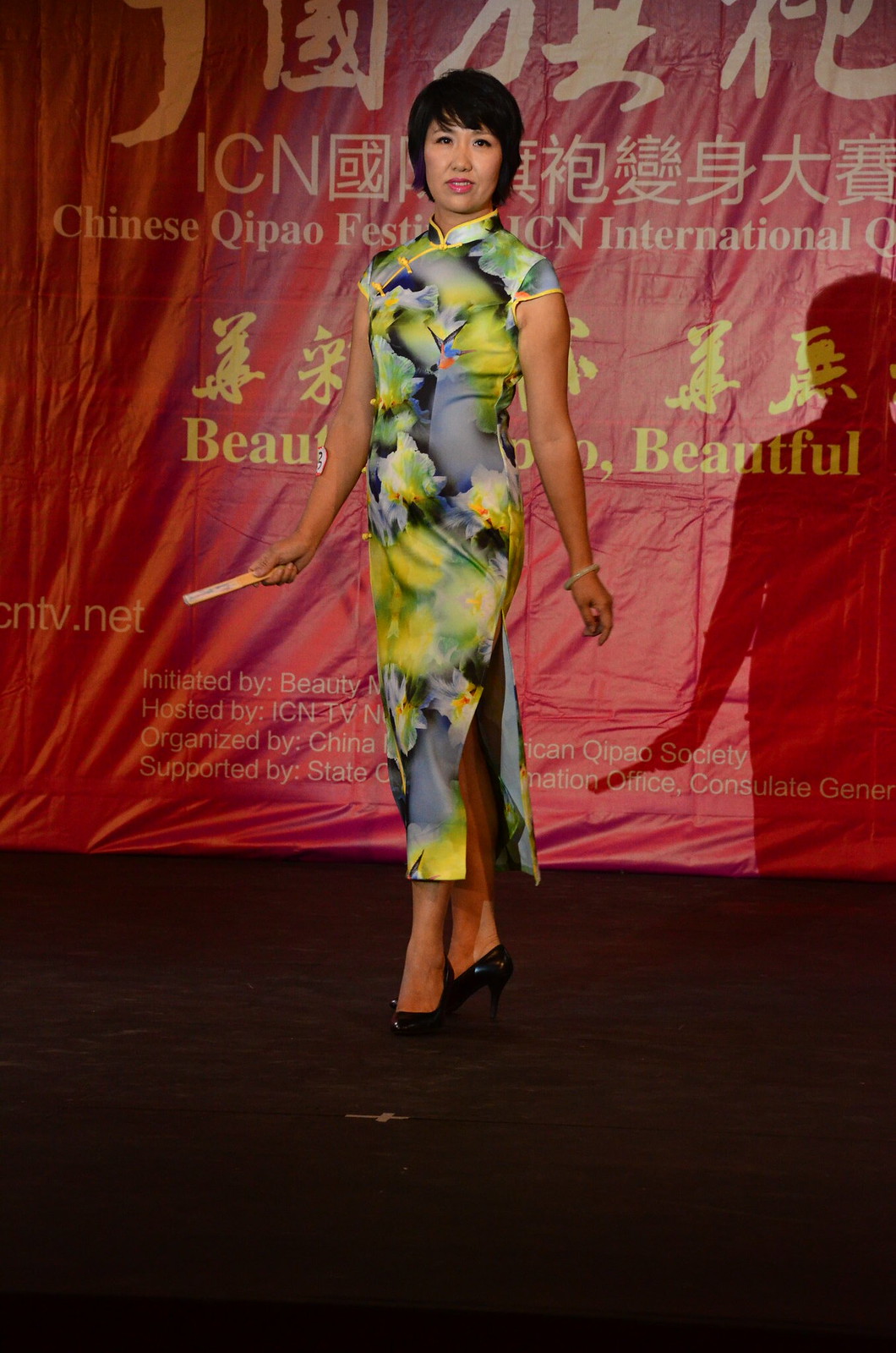The image depicts a woman with short dark hair, standing on a stage with a black floor and a wrinkly red fabric backdrop. She is wearing a green floral cheongsam dress that features a high slit on the right side, extending up to her hip or thigh. Her pose is poised with her weight on her rear right foot and her left foot forward. Her arms are extended at her sides, with a silver bracelet adorning her left wrist and a folded paper fan held in her right hand. The woman is smiling directly at the camera. The backdrop includes a projection on the left corner, and to the right, it displays text that reads "ICN Chinese Qibao International" along with Chinese characters. The setting appears to be indoors, likely during a festival or awards show, indicated by the decorative elements and the particular arrangement of the stage area. There is a tape cross on the floor to mark her spot, emphasizing the precision required for stage presentations. The image captures an atmosphere filled with vibrant colors including black, red, yellow, off-white, green, tan, and gray.